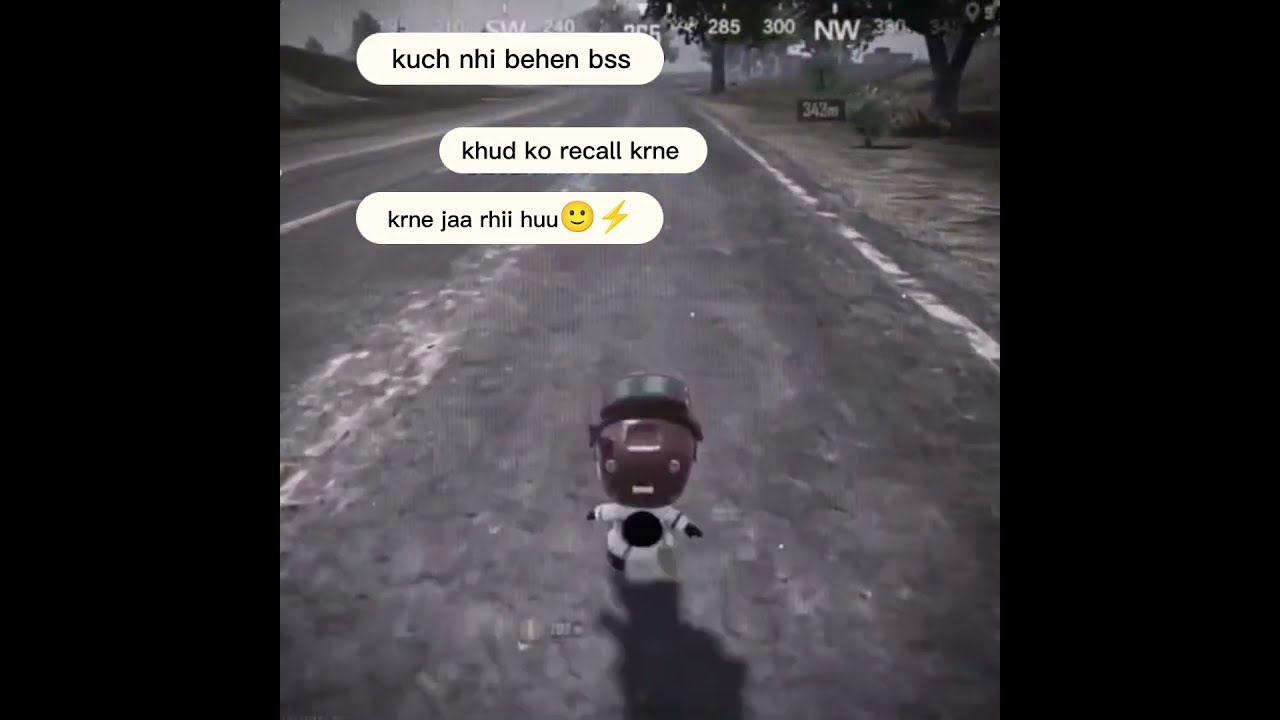In the foreground of this image, which seems to be from a video game with a surreal, cartoonish style, we see a peculiar humanoid character positioned on a gray, hand-drawn road with white lane markings. This character, akin to a cartoon avatar, has an unusually large, brown metallic head adorned with a small, green circular cap. Its eyes resemble tiny beads or buttons, spaced widely apart with no visible nose. The mouth is a thin, white horizontal rectangle, giving it a simplistic, almost abstract appearance. It wears an outfit resembling astronaut gear, featuring a white long-sleeved top with a black circle in the center and white pants, while its hands and feet are brown. A shadow is cast in front of the character, suggesting a light source from behind. The background of the scene is gray, with a misty sky and a few cartoon-esque trees with green foliage and dark gray trunks. Above the character, three white speech bubbles contain foreign text: "kuch mi venen bss," "khud ko recall karne," and "karne jaa rhi hu," accompanied by a smiley face and a lightning bolt emoji. The top of the image resembles a compass with coordinates labeled southwest 240, 265, 285, and 300, northwest, stretching from the top left to the top right. The screen is flanked by blacked-out sections on both sides, focusing the view on the central scene.